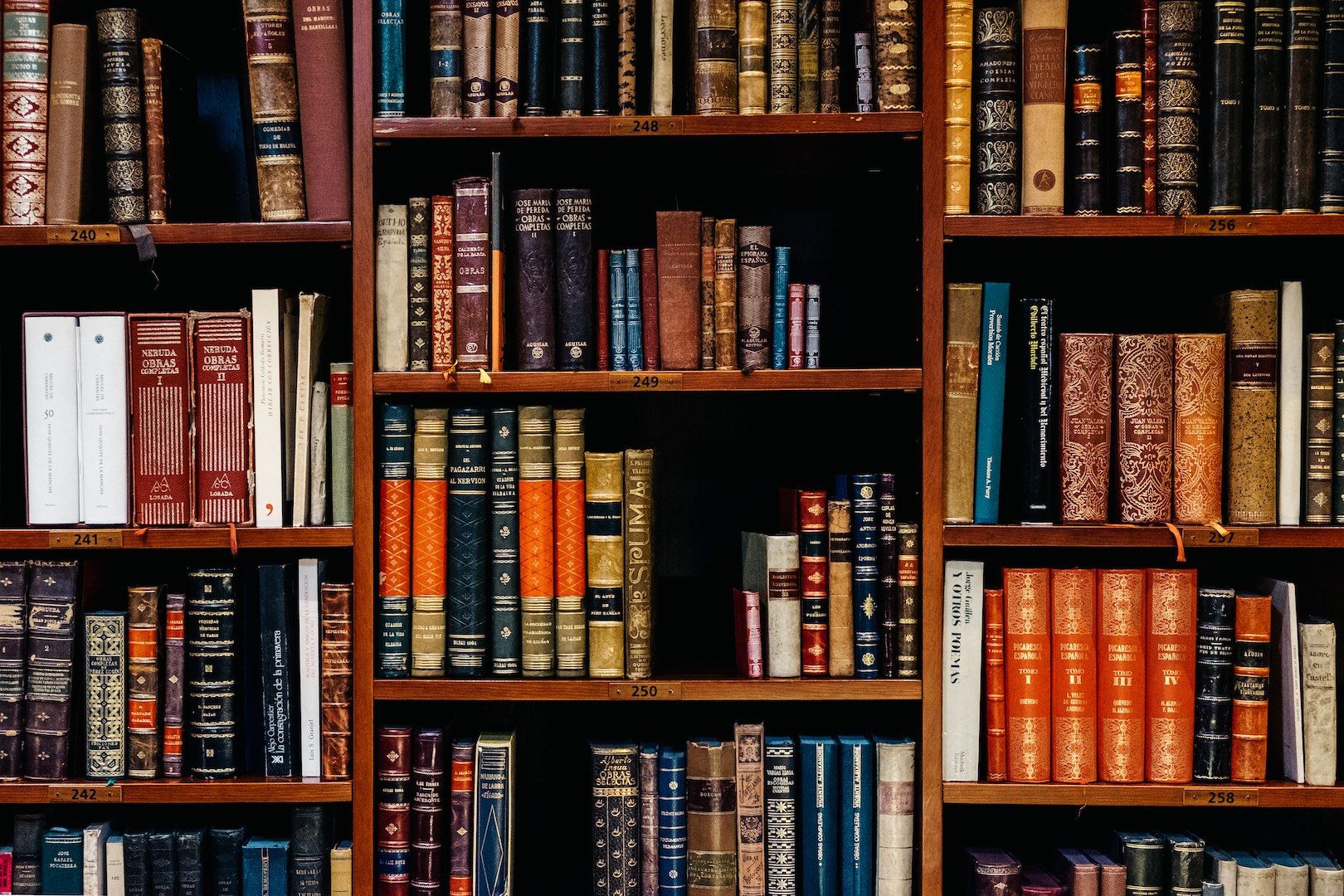The image depicts a close-up view of a partially filled bookshelf, showcasing four layers of classic, hardback-bound books in an array of muted, dark shades including black, brown, blue, burgundy, and tan, with some touches of orange and gold gilt embellishments. The books vary between older classics and a few reference titles, and several empty spots suggest that some books have been recently taken out for reading. The bookshelf is made of medium to dark brown wood, with each shelf bearing a small plate with black numbers, with the left rows marked 240 to 242, the middle from 248 to 250, and the right from 256 to 258. This composition, possibly situated in a private study, exudes an inviting and elegant atmosphere perfect for browsing and discovering literary treasures.